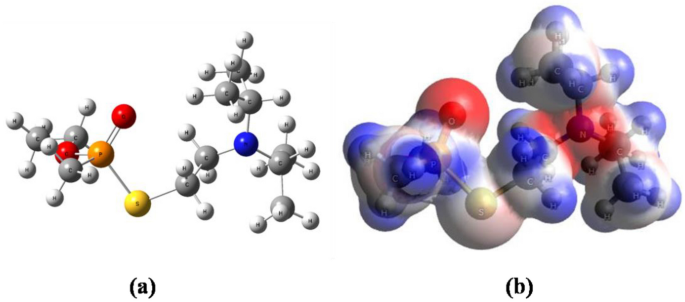This illustration appears to be a scientific diagram, likely from a structural chemistry textbook, depicting molecular structures. The image is divided into two sections, labeled A on the left and B on the right. Image A features a detailed 2D assembly of interconnected molecules, portrayed in various colors: phosphorus atoms in yellow or orange, hydrogen atoms in white, carbon atoms in grey, nitrogen atoms in blue, and sulfur atoms in red. Image B depicts a similar arrangement of molecules but rendered in a 3D perspective. This 3D depiction shows the same molecules as in Image A, with the key difference being that they are enveloped in a transparent, bubble-like structure, suggesting an environmental interaction, possibly with water molecules. The intricate representation highlights the spatial and interactive dimensions of the molecular structures.